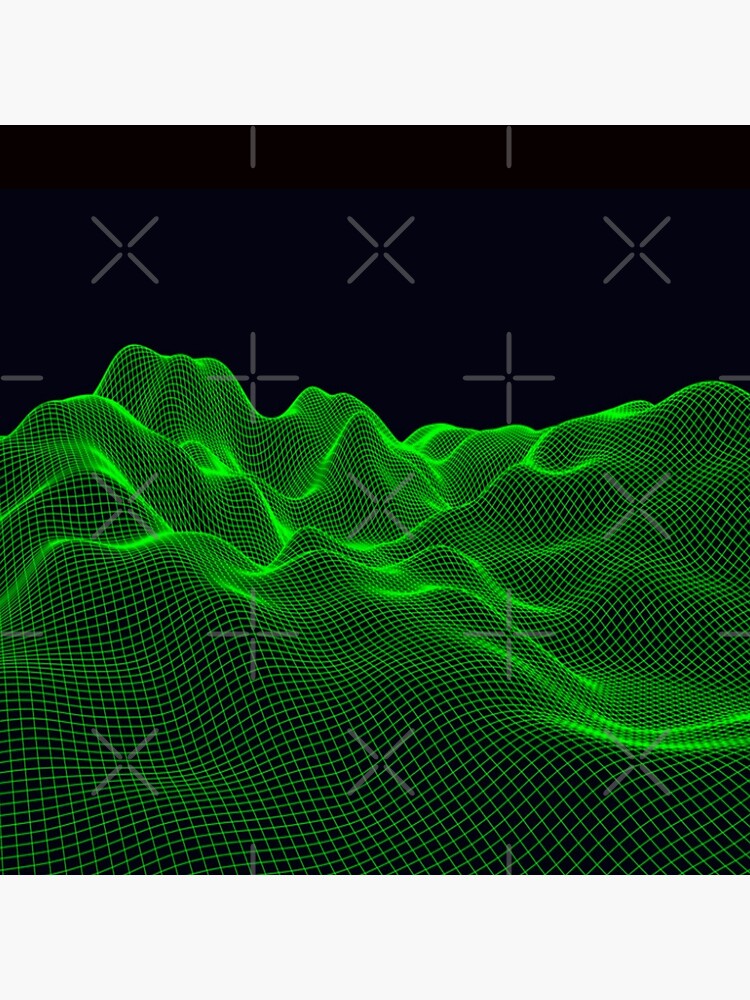The image is a detailed computer-generated 3D rendering of a grid surface resembling a mountainous landscape. The surface is composed of several interconnected peaks and valleys, creating a visually rich terrain. The mountains are depicted in various shades of green, progressing from a bright green at higher elevations to a darker green at the base, mingling with the black background.

A distinct overlay of plus and X symbols, resembling a watermark or rangefinder marks, is uniformly distributed across the image, adding a sense of structure and measurement. Overall, the composition has an artificial, almost holographic quality, enhanced by the bright fluorescent lime green hues reminiscent of some sci-fi aesthetics. The background of the entire image is solid black, which contrasts sharply with the vivid green of the grid-rendered terrain.